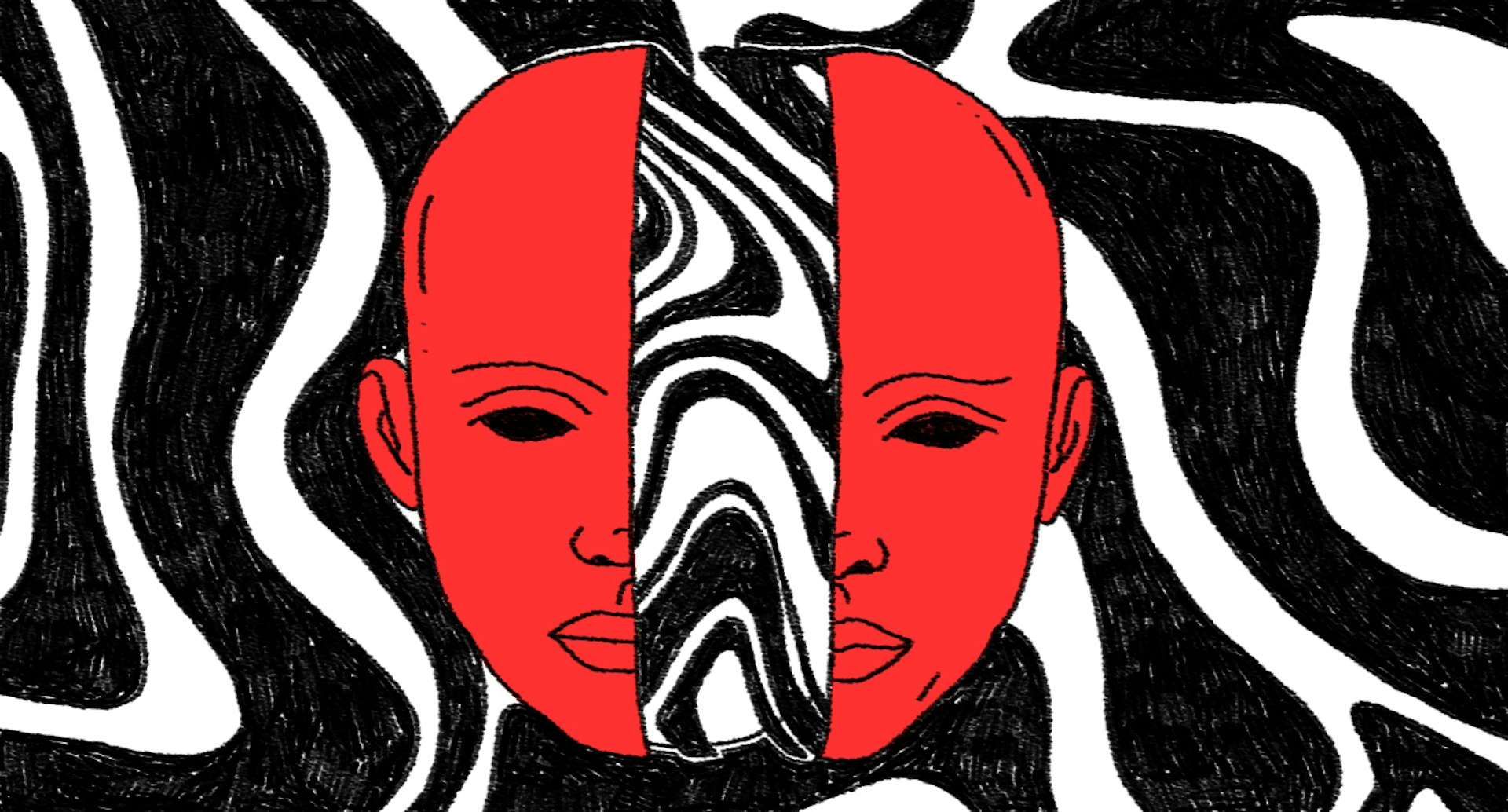This artwork is a detailed drawing, possibly created with pen, featuring a prominent red human face that is split vertically down the middle. The face, which appears to be that of a child, is characterized by its striking red skin and dark black eyes. The lack of hair emphasizes the stark features. The split in the face reveals a gap filled with undulating black and white squiggly lines, reminiscent of zebra stripes, that flow through the center like a swirling river. These black and white wave patterns extend across the background and flank either side of the disjoined face, enhancing the visual impact of the piece. The overall composition is confined within a rectangular frame, suggestive of a banner, graphic, or logo, and presents a compelling interplay between the vivid red of the face and the monochromatic undulations surrounding it.